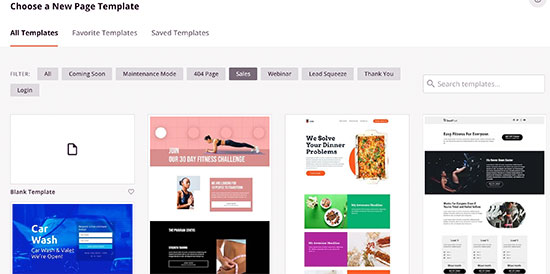This is a detailed caption of a screenshot of a web page dedicated to selecting a new page template. In the upper left corner, there is the heading "Choose a New Page Template." Below this heading, there are three tabs labeled "All Templates" (highlighted), "Favorite Templates," and "Saved Templates" (both not highlighted). Beneath these tabs are horizontal filter categories like "All," "Coming Soon," "Maintenance Mode," "404 Page," "Sales," "Webinar," "Lead Capture," "Squeeze Page," "Thank You," and "Log In." To the right of these filters is a search bar for finding specific templates.

Underneath this search bar, on the right side of the screen, there are template options displayed. One notable template is a white rectangular icon featuring a small paper symbol in the center. Next to this is a visually engaging pink rectangle with the text "Join Our 30-Day Fitness Challenge," accompanied by an image of a person doing push-ups. To the right of these template options, there is another template with the heading "We Solve Your Problem," encapsulating the essence of the offerings with a full-page design.